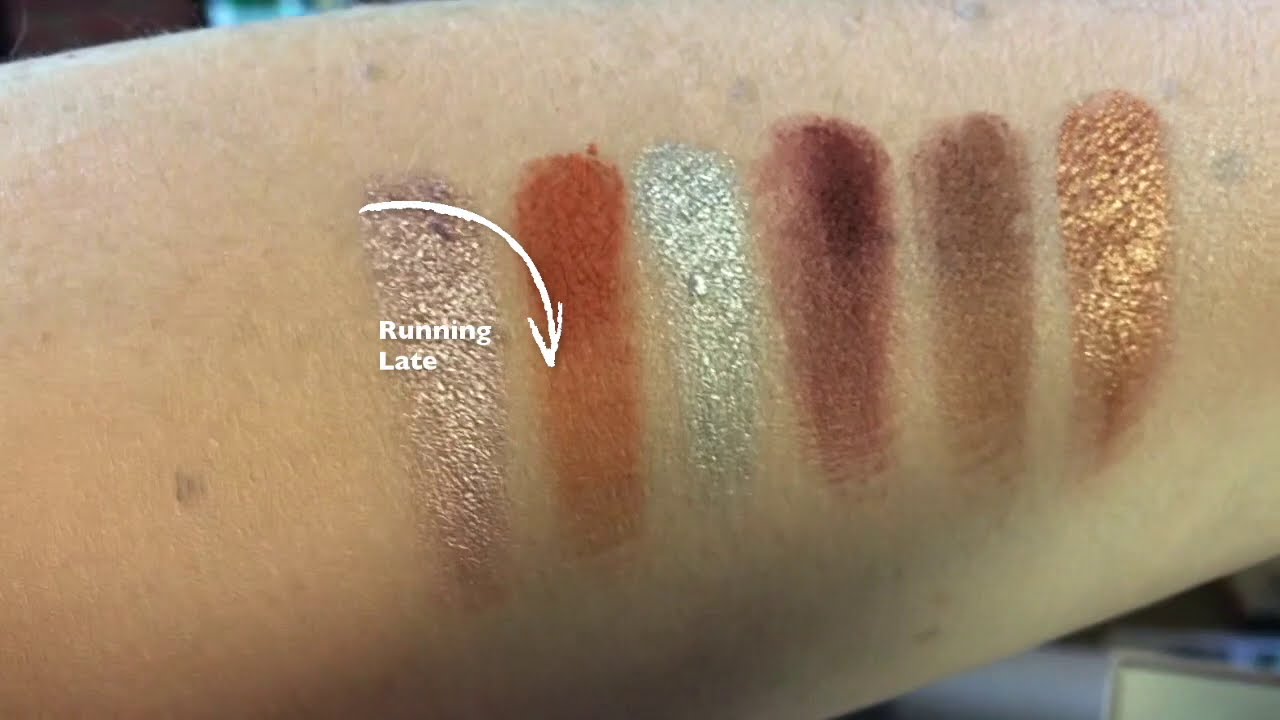The image features the forearm of a white person, prominently displayed horizontally from left to right. The arm is dotted with what appear to be age spots, distributed from the left side to the upper and right side. Six vertical streaks of makeup samples traverse the forearm, each showcasing different colors. The first streak is a sparkling gold with the phrase "Running Late" written in white letters; the words "Running" and "Late" are vertically aligned. An arrow starts above this gold streak, curves to the right, and then swoops downward, pointing towards the second streak. This second streak is an amber or rust color. Following this is a silver-colored streak. Next is a streak of maroon or purple, then a medium brown streak, and finally a bright, shiny gold streak. The background of the image is dark in the corners, except for the bottom left, which might feature part of a table or some indistinguishable structures.